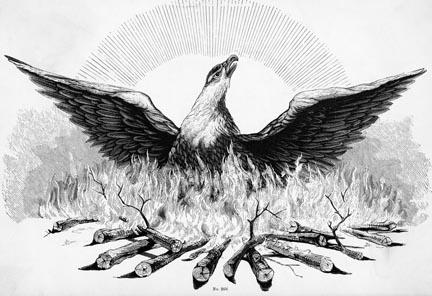This black-and-white, pencil-drawn image features a majestic eagle with its wings fully spread, appearing to gaze intently towards the sky. The illustration captures the eagle with its top chest and neck highlighted in white, contrasting against its black wings, which are subtly detailed with white edges to distinguish the feathers. Rising behind the eagle, arcs of lines create a backdrop reminiscent of a sunrise or sunset. The lower half of the eagle's body is obscured by a roaring fire, with swirling flames engulfing the area. Surrounding the fire are scattered logs, arranged in a circular pattern that evokes a traditional campfire, reminiscent of a classic Boy Scout setup. Dark smoke billows from the sides of the flames, adding to the dramatic and intense atmosphere of the scene. All elements in the drawing are rendered in varying shades of gray, emphasizing the stark contrasts and intricate details of this compelling and dynamic composition.